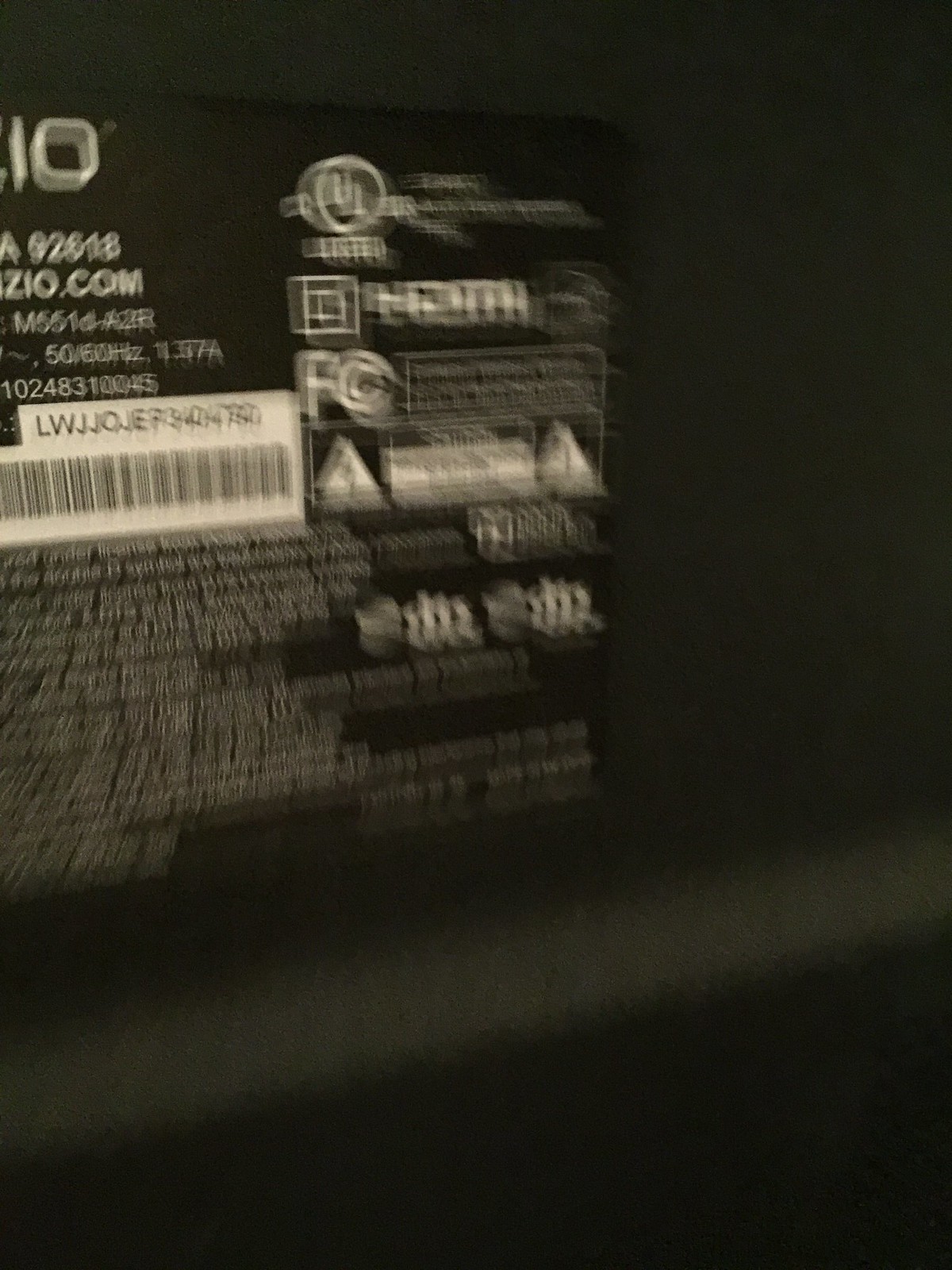The image depicts the back of a black electronic device or battery. The focal point is a label that stands out against the darker black background of the device itself. The entire image is slightly blurred, making it challenging to read the finer details. However, the label clearly has white lettering and a prominent barcode, accompanied by a long serial number above it. Beneath the barcode, there are multiple lines of smaller text interspersed with larger words, though the blur prevents full clarity. Among the discernible text elements, "UL" and a word resembling "tested" can be vaguely identified, suggesting some form of certification or compliance. The overall appearance indicates standard labeling for electronic equipment.